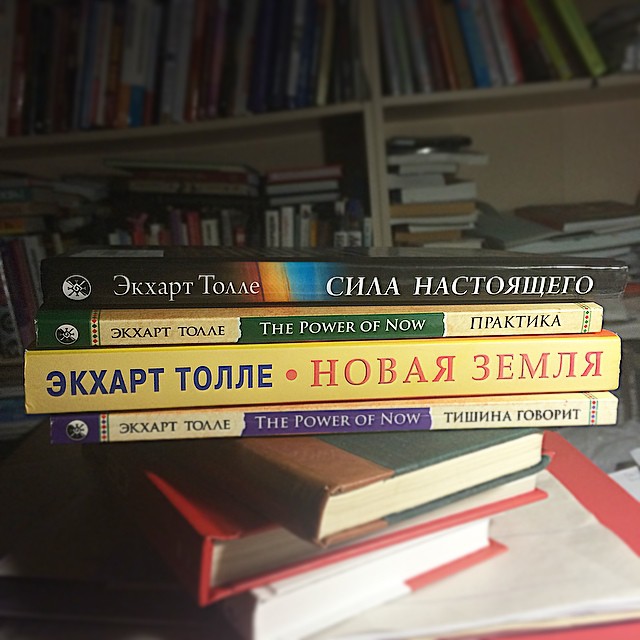The photograph depicts a cluttered array of books on a table in a dimly lit room, likely an office or a personal study, in front of an overloaded, cream-colored bookshelf. The foreground features a stack of books, with the top four displaying their spines forward. The topmost book is black with white text, showing an eclectic mix of seemingly foreign characters that resemble a different language, possibly Russian, but are actually English letters arranged in an unusual manner. Two of these books, prominently The Power of Now, are visible. One boasts a green and white spine and another a purple and white one. Beneath these lie additional books, turned diagonally with their spines facing left, including a green and brown one, a red one, and others that are partially obscured. Abundant with a variety of colors—yellow, purple, green, black, and beige—the collection appears chaotic and dynamic. The background shows a bookshelf crammed haphazardly with more volumes, some standing upright, others piled horizontally, contributing to the scene of an avid reader's or academic's unkempt yet vibrant environment.